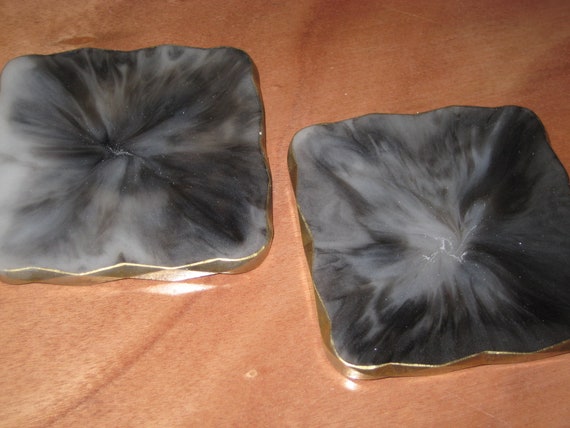The photograph captures a sleek wooden tabletop or desk with a glossy, resin-like finish, resembling a bar top material. Resting on this surface are two square crystal coasters, each approximately half an inch thick. These coasters feature a marbled black and white pattern that radiates from the center outward, akin to the inner look of a quartz rock. Their edges exhibit slight scalloping, giving them an imperfect square shape with added texture. Each coaster is bordered by a gold-plated rim adorned with subtle triangular markings. The left coaster displays a lighter pattern compared to the darker right one, highlighting their unique yet complementary designs.